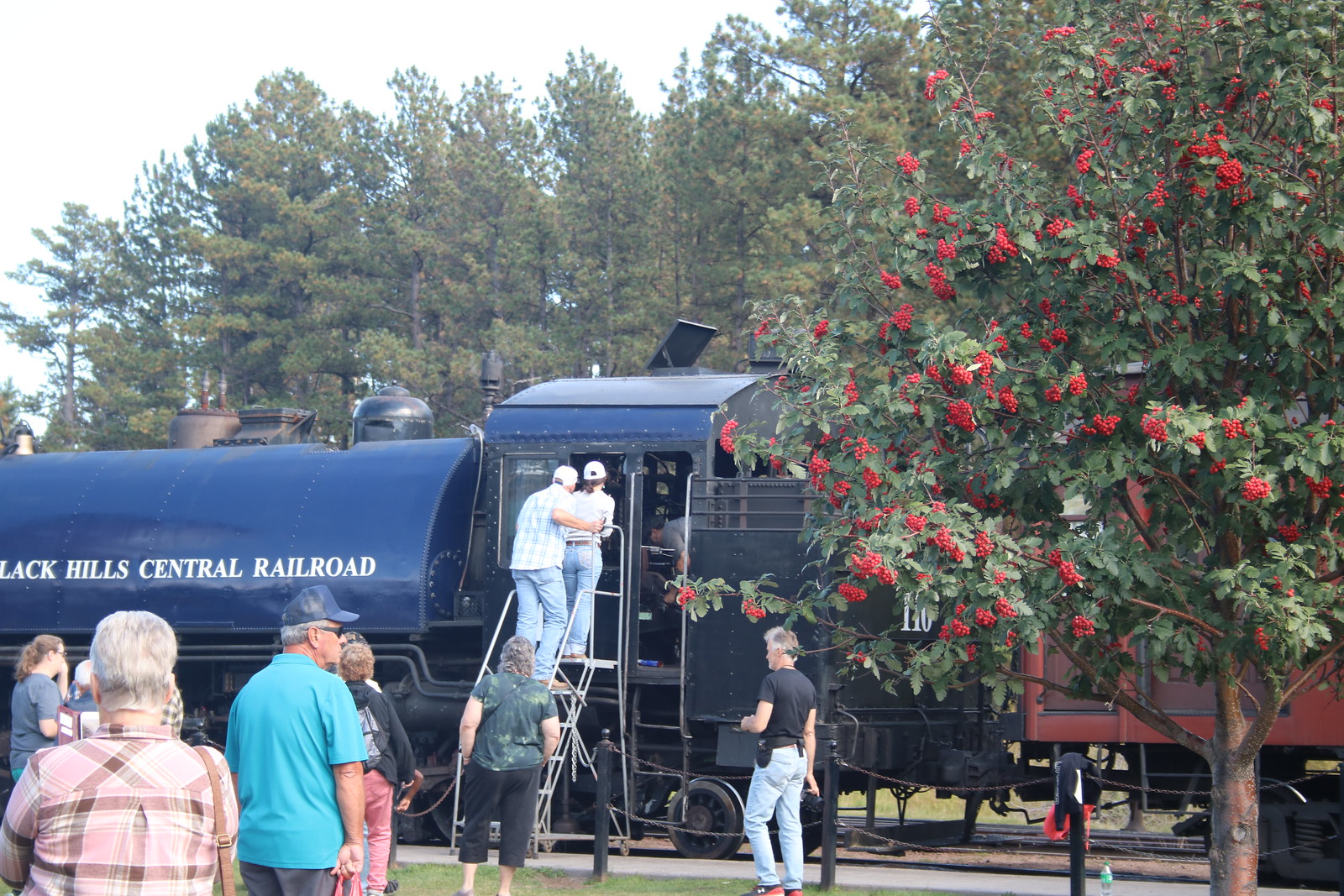Captured on a bright and clear summer day, this outdoor photo showcases the Black Hills Central Railroad train, stationed prominently in the foreground. The train, with its distinctive blue front emblazoned with the name "Black Hills Central Railroad," stands as the focal point amidst a vibrant scene. A line of people eagerly waits to either exhibit, watch, or ride the train, hinting at a possible event or a journey about to commence. To the right, a lush green tree adorned with red berries partially obscures the train. In the background, tall trees rise against a vivid blue sky, adding to the picturesque setting. The scene captures a mix of anticipation and natural beauty, with the crowd's excitement and the train poised for adventure.